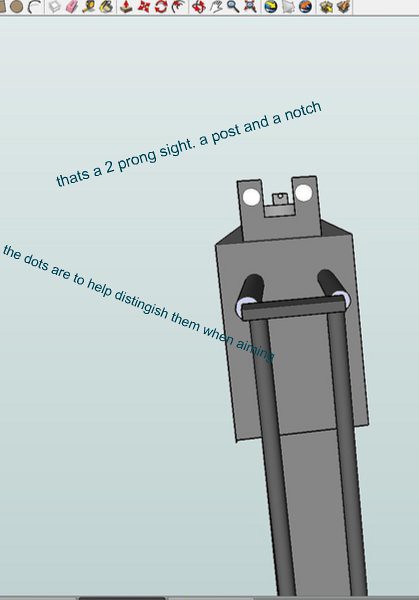This portrait-oriented image appears to be a screenshot from a video game tutorial. A light gray header spans the top, populated with various small, blurry icons resembling emojis or tool representations: a brown rectangle, a brown circle, a letter C, a white box, a pink eraser, a yellow tape measure, additional yellow and red items, a red person on a box, a red throwing star, a refresh button, an indeterminate red object with black extensions, a hand, a magnifying glass, a compass, a circle with a yellow arrow, a white map, a circle with an orange star, and indistinct boxes with yellow and orange details. Beneath this header, two lines of text in teal and dark blue appear diagonally against a pale aqua background. The top line reads, "That's a two-pronged sight, a post and a notch," while the second, partially obscured line states, "The dots are to help distinguish them when airing." Dominating the lower half of the image is a dark gray metal structure with two vertical bars leading to a lighter gray rectangular shape resembling a robotic figure, with a U-shape on the top adorned with two white circles resembling eyes, further enhancing the visual elements of this screenshot.